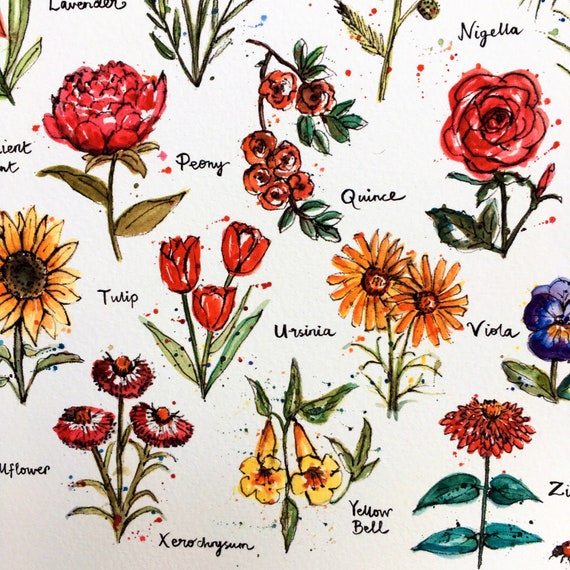This image portrays an artistic hand-drawn pattern on what appears to be a white canvas, potentially designed for a cloth item like a tablecloth. The pattern features a variety of vividly colored flowers, such as peonies, quinces, tulips, violas, sunflowers, zinnias, nigellas, lavenders, and yellowbells. Each flower is carefully illustrated in its true-to-life colors, accented by accompanying leaves and sprigs. The names of the flowers are elegantly written in cursive beside their respective illustrations. The arrangement is scattered across the canvas without following any specific alphabetical order. The overall effect is highly detailed and visually appealing, possibly rendered in watercolor, as evidenced by some paint splatters that lend a unique artistic touch to the piece.